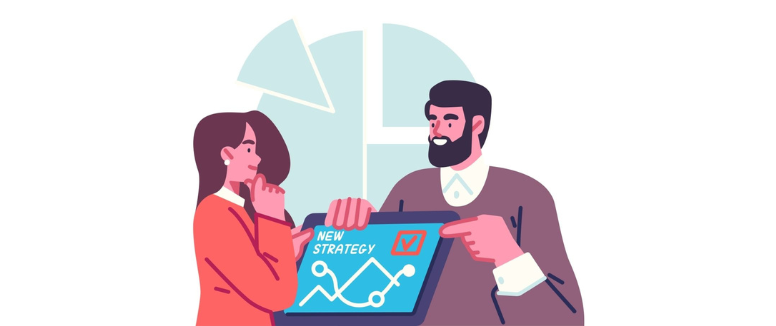This is a cartoon-style digital image featuring two individuals, a man and a woman, set against a white background. The woman, positioned on the left, is light-complected with brown hair and is wearing an orange shirt over a white undershirt, adorned with white stud earrings. She is depicted contemplating with her right hand on her chin while her left hand holds a tablet. The tablet displays the text "NEW STRATEGY" in white lettering, accompanied by an orange square with a checkmark and a white graph featuring a V-shaped line at the top.

The man standing beside her is taller, with a beard, dark hair, and a brown mustache. He is dressed in a brown jacket with a visible white undershirt and is smiling while pointing at the orange checkmark on the tablet. In the background, there is a cyan pie chart, showing half of the pie and two quarters – one floating closer and the other farther away. Additionally, a floating triangle is visible to the left of the pie chart. The overall composition suggests a collaborative brainstorming or planning session between the two characters.